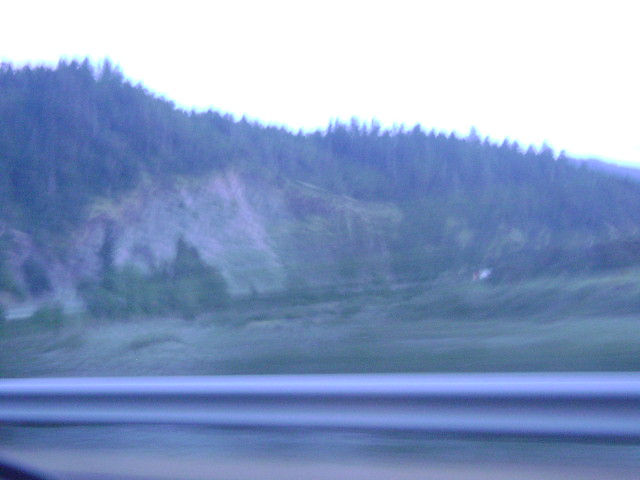This daytime landscape photograph, taken from within a car, showcases a verdant hillside densely covered with lush green trees. The scene is bathed in ample sunlight under a clear, pale blue sky adorned with soft white clouds. A metallic guardrail is visible in the foreground, indicating the vantage point from a roadside or highway. In certain areas of the hillside, evident scars suggest previous mudslides, exposing patches of barren earth amidst the thriving foliage.